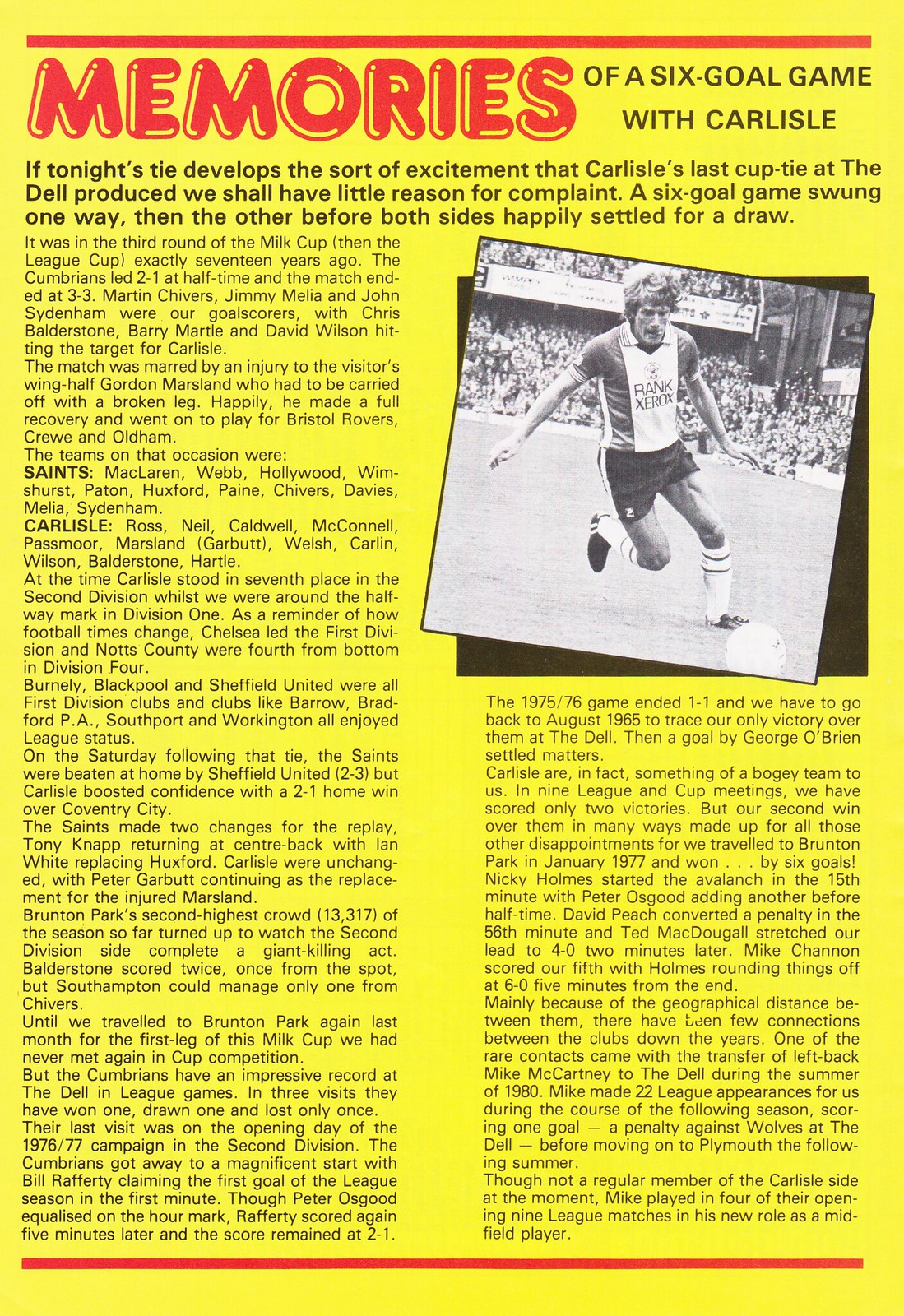The image depicts a scanned page, likely from a magazine, showcasing a yellow-background article titled "Memories of a Six-Goal Game with Carlisle." The title is prominently displayed at the top in unique, uppercase red font with a red line above it. Beneath the title, the article features a black-and-white photograph of a soccer player with a crowd in the double-decker bleachers behind him. The player, who has light, floppy hair, is about to kick a ball on a field or stadium. He is wearing a short-sleeved shirt, dark shorts, long socks up to his knees, and black cleats, with "Rank Xerox" printed on his jersey. The article text includes a blurb: "If tonight's tie develops the sort of excitement that Carlisle's last cup tie at the Dell produced, we shall have little reason for complaint as six-goal games swung one way, then the other, before both sides happily settled for a draw." Additional paragraphs follow beneath this blurb, with another red line marking the bottom of the page.